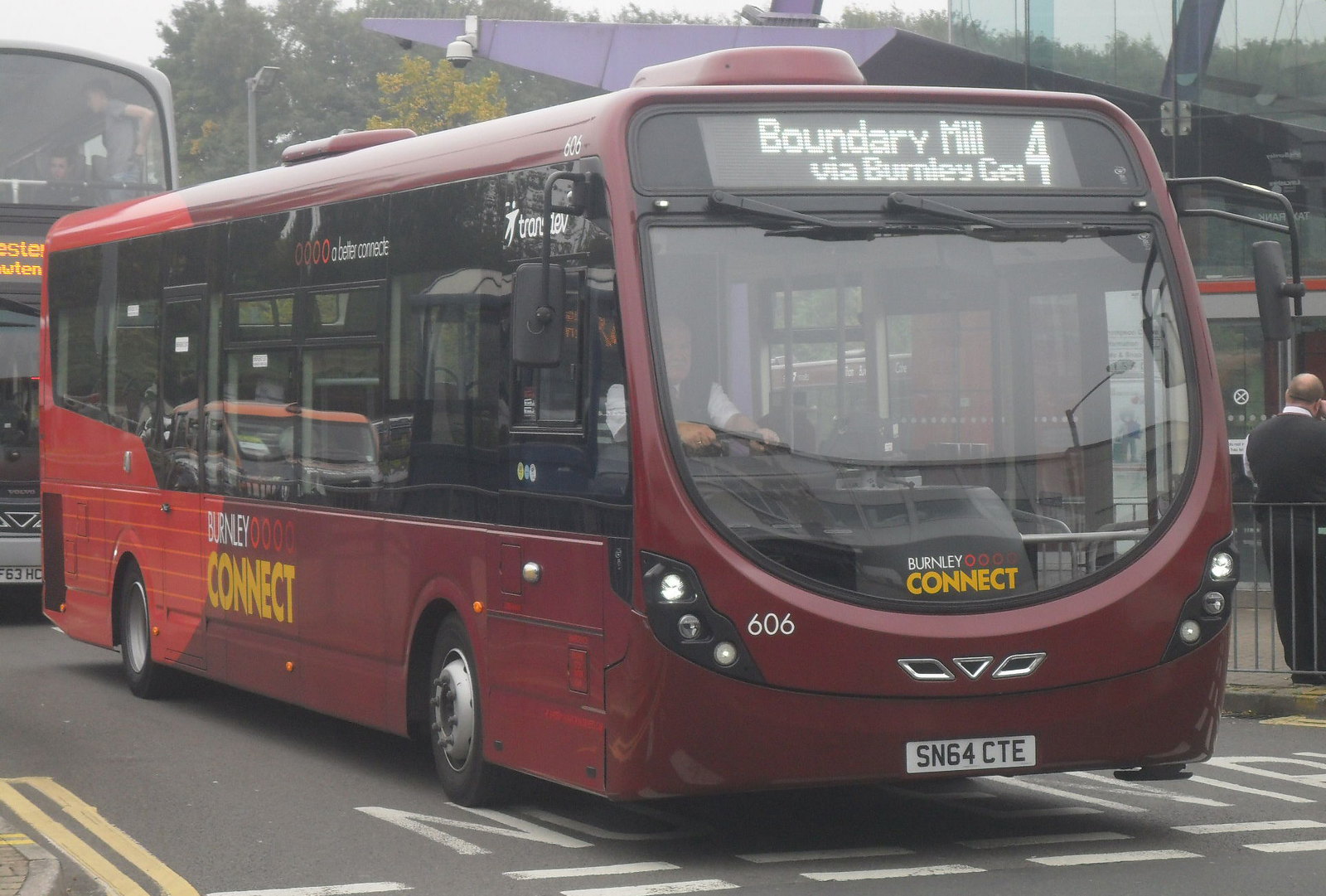In this vibrant, outdoor scene, a predominantly red and dark purple bus dominates the frame. The front of the bus features the number "606" along with the inscription "Burnley Connect," while its digital sign at the top reads "Boundary Mill via Burnley GE." The rest of the text on the sign is partially cut off, likely due to the moving display, and it includes the route number "4". The bus, adorned with the license plate SN64CTE, appears to be a double-decker similar to those commonly seen in London, despite having elements distinct to the Burnley area. The surrounding setting includes trees and natural light, contributing to a bright backdrop. Another bus is visible in the rear, though partially cut off, indicating a possible bus depot in the vicinity. A man stands on the right side of the image, enriching the lively atmosphere of this street scene.